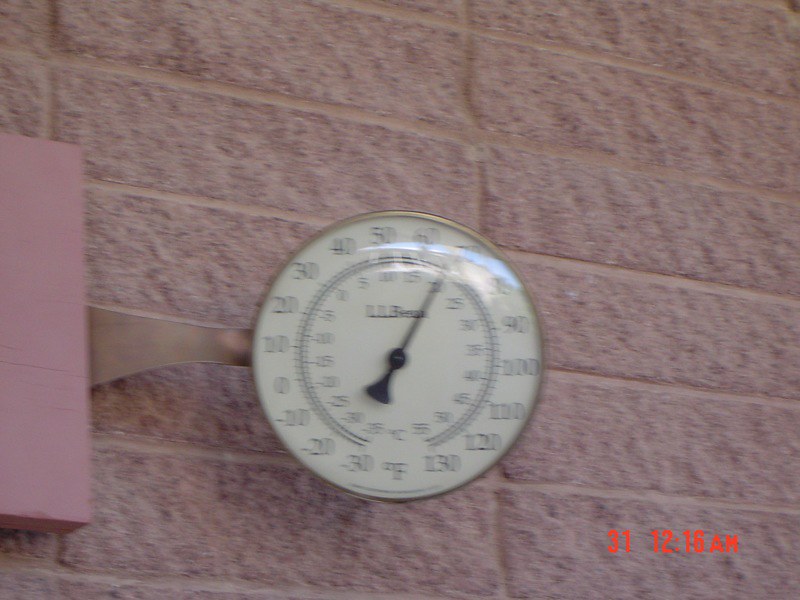The image depicts a temperature gauge or thermometer mounted on a red brick wall. The thermometer features a brass outer frame and a brass mounting bracket that connects to a red box, securing it to the wall. The circular design of the thermometer includes a white face with black numerals ranging from -30 to 130 degrees. The face is protected by a clear glass cover, which has a slight glare. The center of the dial prominently displays the brand name "L.L. Bean" in black lettering, though the photo is somewhat blurry. A black needle indicates the temperature, which appears to be around 68 or 69 degrees Fahrenheit. Additionally, a red timestamp in the lower right-hand corner of the image reads "3-1 12:16 a.m."